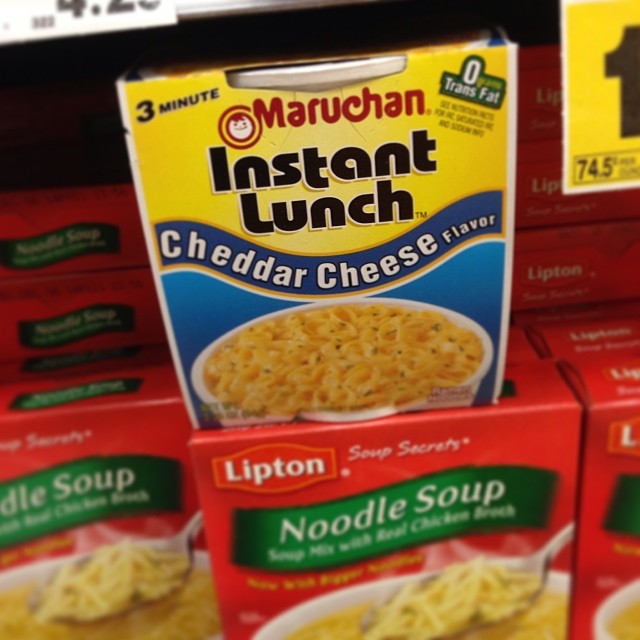A close-up of a supermarket shelf showcases prominently a box of Lipton's Soup Secrets Noodle Soup. The red packaging features a green, curvy banner across the top with "Noodle Soup" written in white letters. Below the banner, there's an enticing photo of a white bowl filled with steaming hot noodle soup, looking more delicious than one might expect the actual product to be. A spoon loaded with noodles is positioned invitingly above the bowl, adding to the soup's appeal. Several of these boxes are both upright and stacked on their sides, creating a neat display.

Among these neatly arranged boxes, an out-of-place instant lunch cheddar cheese flavor cup catches the eye. Its appearance suggests that it was likely discarded by an indecisive shopper who was swayed by the allure of the Lipton Noodle Soup. The instant lunch cup, which looks less appetizing in comparison, boldly advertises its 0% trans fat content and promises a quick three-minute cooking time. Its haphazard placement disrupts the uniformity of the noodle soup display.